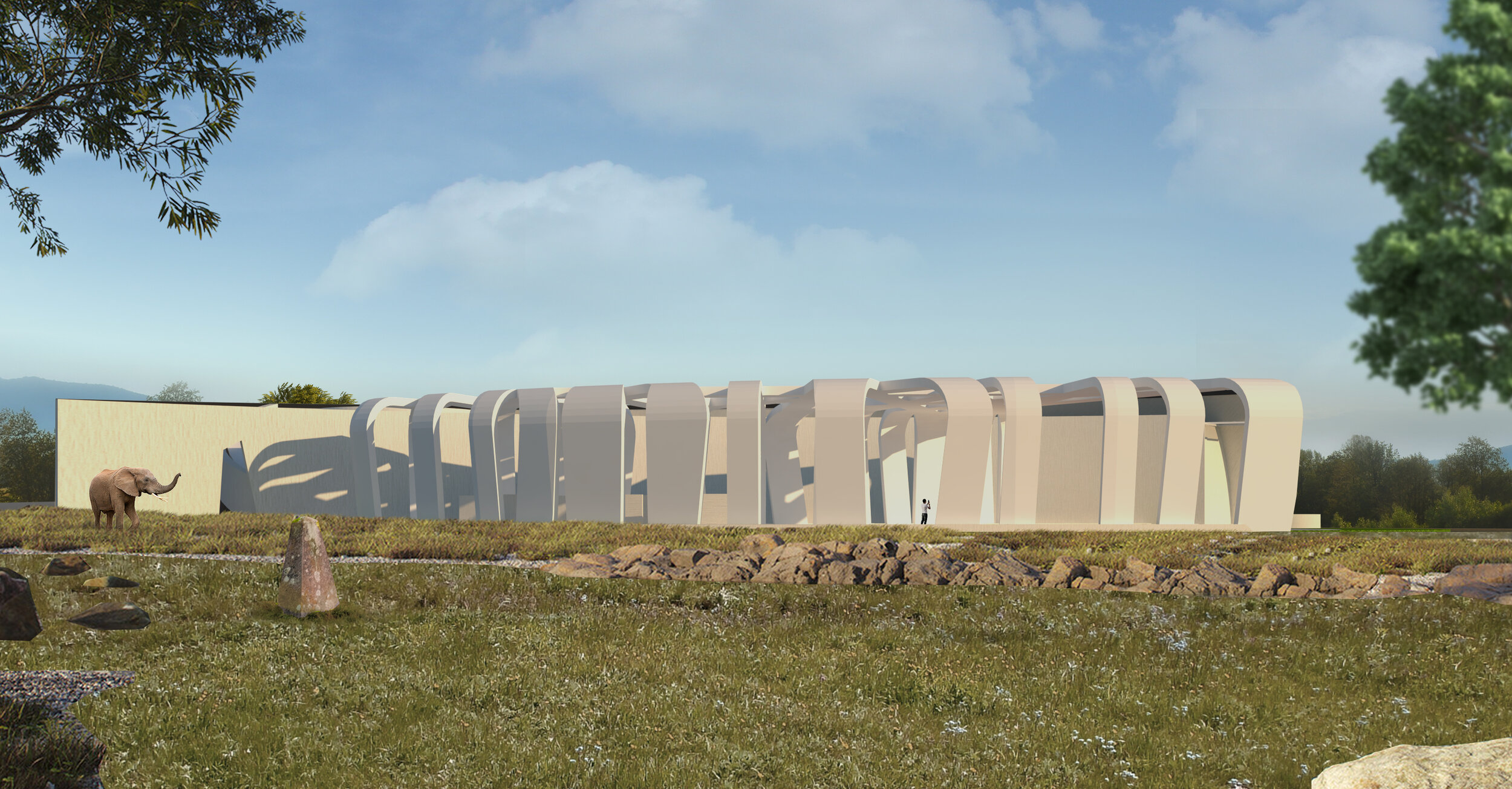In the foreground of this detailed horizontal nature scene, we see a large, one-story structure with an intricate design. The white building has several curved strips that meet at the top, creating open spaces in between, almost resembling an upside-down clothes basket. This seems more like an art installation or sculpture rather than a functional building. To the left of this sculpture, there is an elephant, possibly a baby elephant, adding an intriguing element to the setting. A person is seen underneath, seemingly taking pictures of the structure. 

The background reveals a powder blue sky dotted with clouds, framing the scene in a gentle light. To the right and left, trees punctuate the landscape, while mountains stand tall in the far distance. In the center foreground, there's a grassy expanse interspersed with rocky areas, and it appears there's a creek or stream meandering through the rocks. This layered and complex composition combines natural elements with human-made artistry, creating a captivating juxtaposition in the serene outdoor environment.